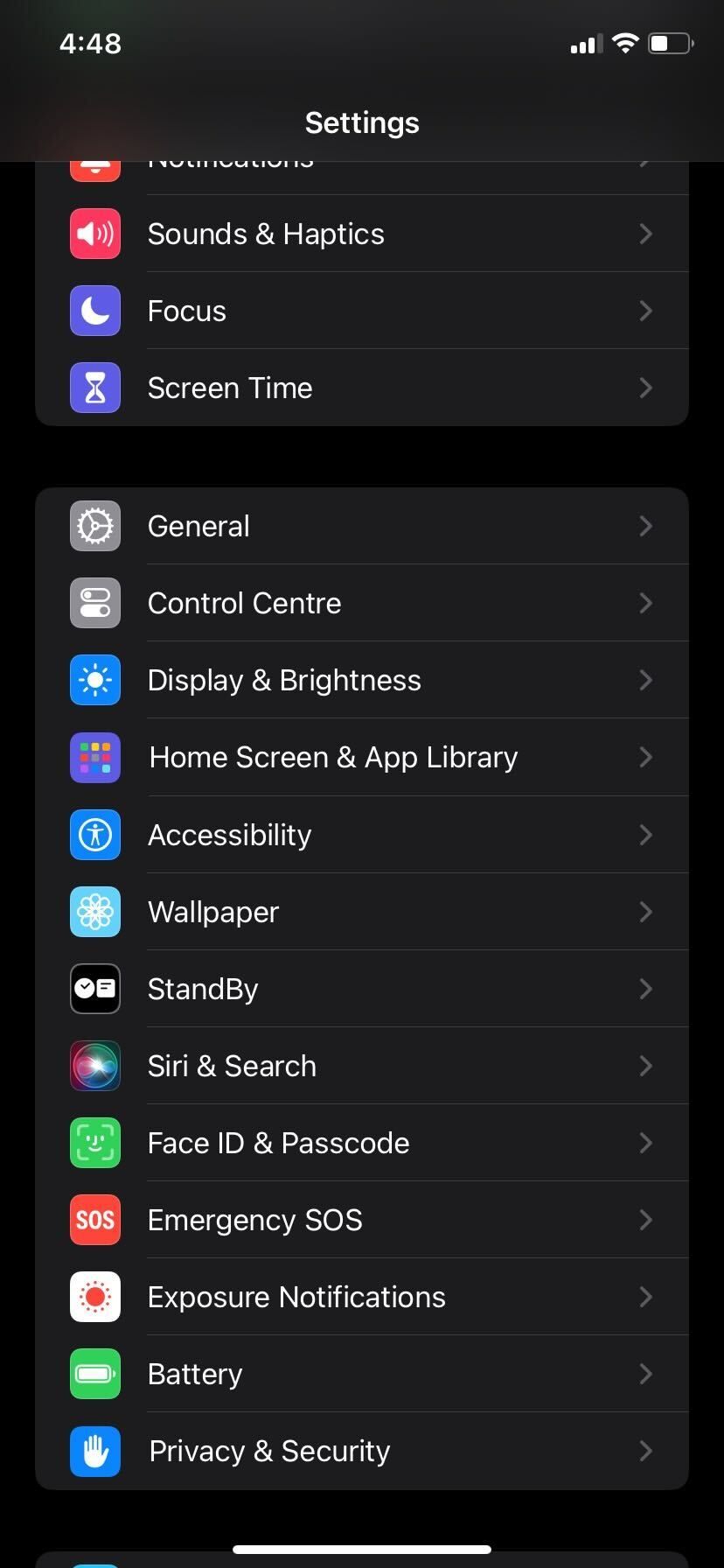This image appears to be a detailed screenshot from a cell phone displaying its settings menu. At the top of the image, the phone's status bar is visible against a black background, showing the time on the far left, followed by icons for signal strength, Wi-Fi connectivity, and battery level to the right.

Just below the status bar, the word "Settings" is prominently displayed. Beneath this title, several settings options are listed in a vertical arrangement, each accompanied by a respective icon. From the top, the visible settings include:

1. **Sound & Haptics** - Represented by a speaker icon.
2. **Focus** - Indicated by a moon icon.
3. **Screen Time** - Depicted with an hourglass icon.
4. **General** - Illustrated with a settings wheel icon.
5. **Control Center** - Shown with an assortment of buttons.
6. **Display & Brightness** - Represented by a sun icon.
7. **Home Screen & App Library** - Depicted with several multicolored squares.
8. **Accessibility** - Illustrated with a human icon.
9. **Wallpaper** - Shown with a flower icon.
10. **Standby**
11. **Siri & Search**
12. **Face ID & Passcode**
13. **Emergency SOS**
14. **Exposure Notifications**
15. **Battery**
16. **Privacy & Security**

Each of these categories is designed to guide the user through various configuration options for their device, from adjusting sound settings to managing privacy and security features. The arrangement is user-friendly and visually structured, facilitating easy navigation through the settings menu.